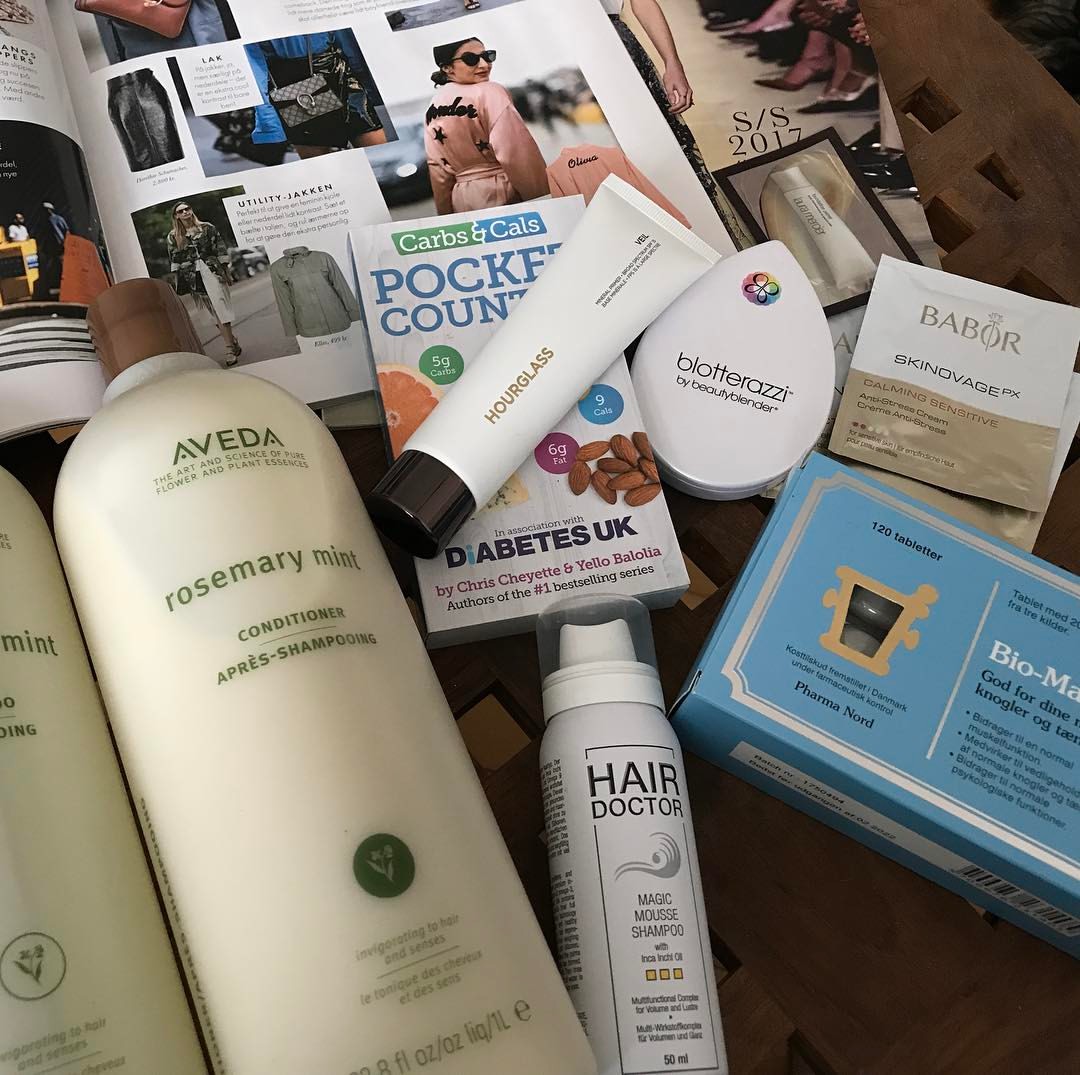On a tan-colored surface, resting prominently in the upper left-hand corner, an open magazine reveals its contents. The left-hand page features a mixture of black printed text and a photograph that occupies half the page, though the subject of the photo isn't specified. Opposite, the right-hand page presents a colorful array of square images showcasing various items. One notable image displays a model clad in a stylish pink coat with black accents. Scattered below and on the magazine are a range of beauty products, including two white bottles with green labels, a white tube with a black cap, and a white aerosol can labeled "Hair Doctor." Among these items, there is also a box labeled "Pocket" something, a blue bar soap box, and two additional cosmetic products, contributing to the assortment of beauty essentials.